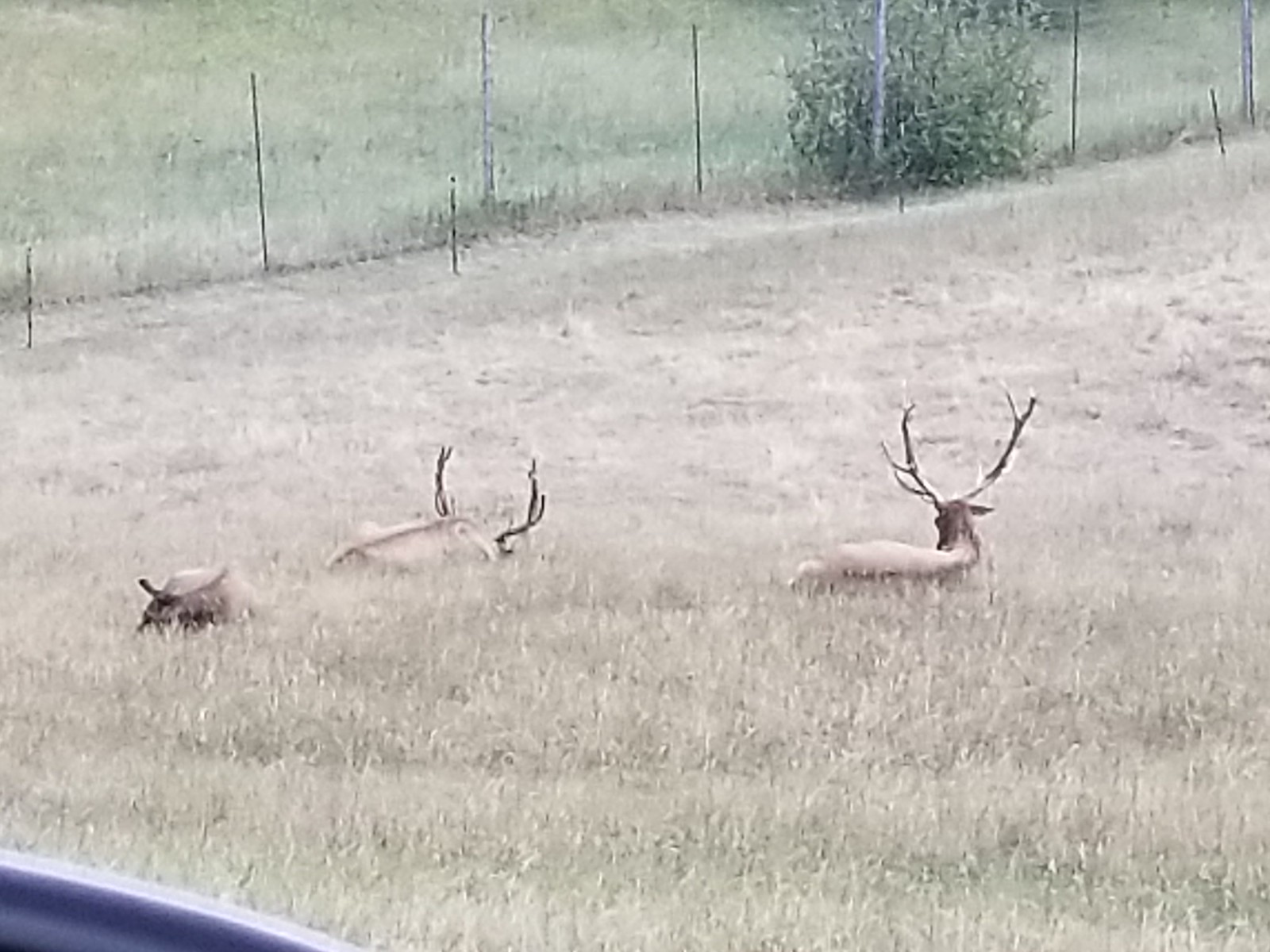This image captures a scene of wildlife featuring three deer resting in a grassy area, possibly within a fenced property that could be a drive-through safari or a hunting reserve. The grass is predominantly brown and dull green, indicating it may be dry or dead. Overhead, we see a high fence demarcating the area, suggesting a controlled environment. 

Centered in the grassy expanse are the three deer. The deer on the far right is oriented away from the camera and is distinguished by its large, pointy antlers. To the left of this deer is another buck, identifiable by its upward-spiking antlers. Further to the left, partially obscured and lying down with its head down, is a smaller deer, possibly a doe, lacking antlers. 

A thin blue strip at the bottom of the image, likely part of a guardrail, adds a hint of color to the otherwise muted landscape dominated by the earthy tones of the grass.